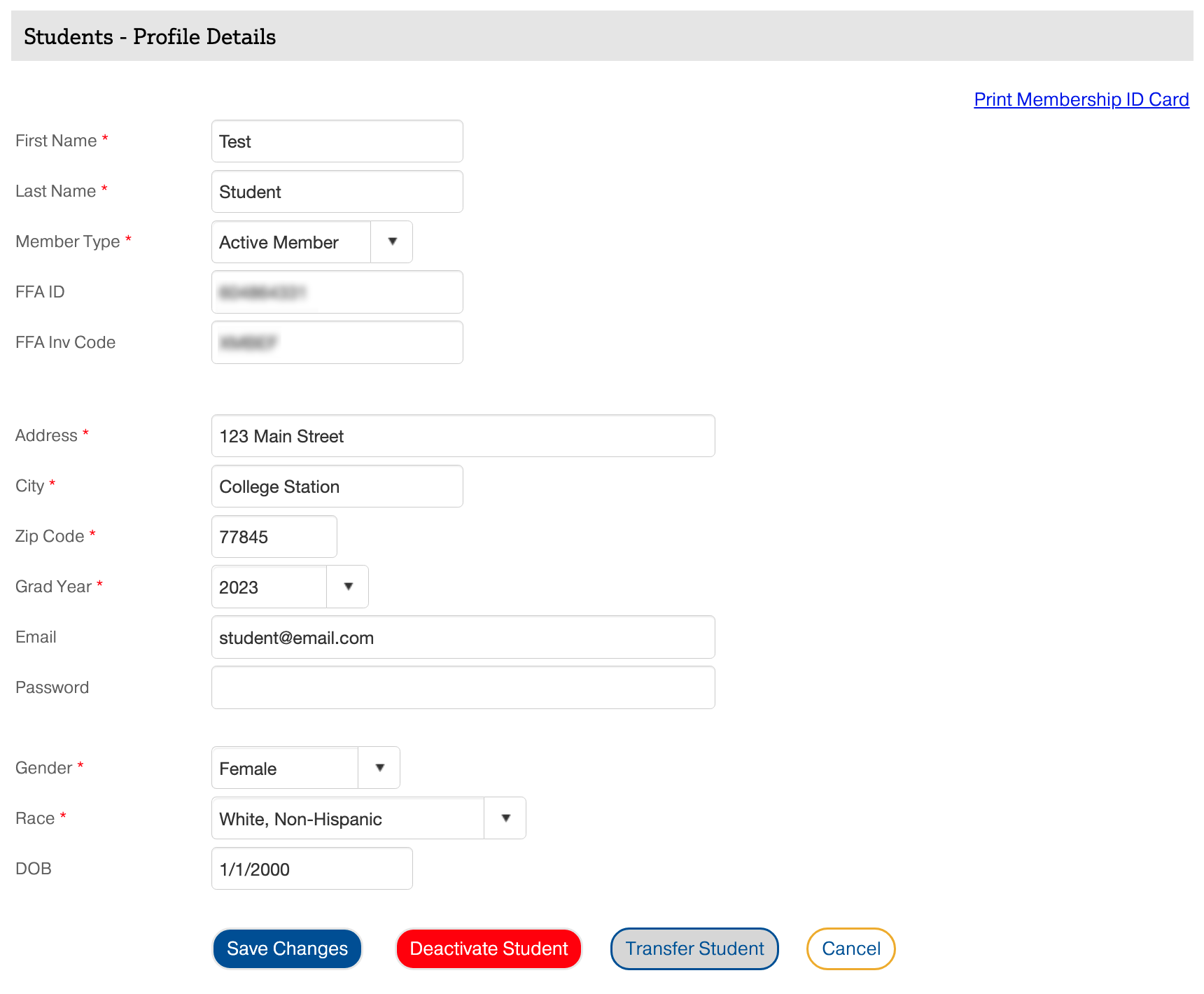This horizontally rectangular image is a screenshot from an information request page. At the top, there's a narrow horizontal light gray banner that reads "Student Profile Details" on the left. On the far right, just beneath the gray banner, is a blue link labeled "Print Membership ID Card."

The left side of the image displays a vertical list of information items beside their corresponding input fields. From top to bottom, the fields are as follows:

- First Name: "Test"
- Last Name: "Student"
- Member Type: "Active Member" (displayed as a drop-down menu)
- FFA ID: Grayed out
- FFA In Vittoria Code: Blacked out
- Address: "123 Main Street"
- City: "College Station"
- ZIP Code: "77845"
- Graduation Year: "2023" (displayed as a drop-down menu)
- Email: "student@example.com"
- Password: (Empty field)
- Gender: "Female" (displayed as a drop-down menu)
- Race: "White, Non-Hispanic" (displayed as a drop-down menu)
- Date of Birth: "01/1/2000"

Along the bottom of the image, there are four buttons aligned side by side:

- A blue button labeled "Save Changes"
- A red button labeled "Deactivate Student"
- A gray button labeled "Transfer Student"
- A white button labeled "Cancel"